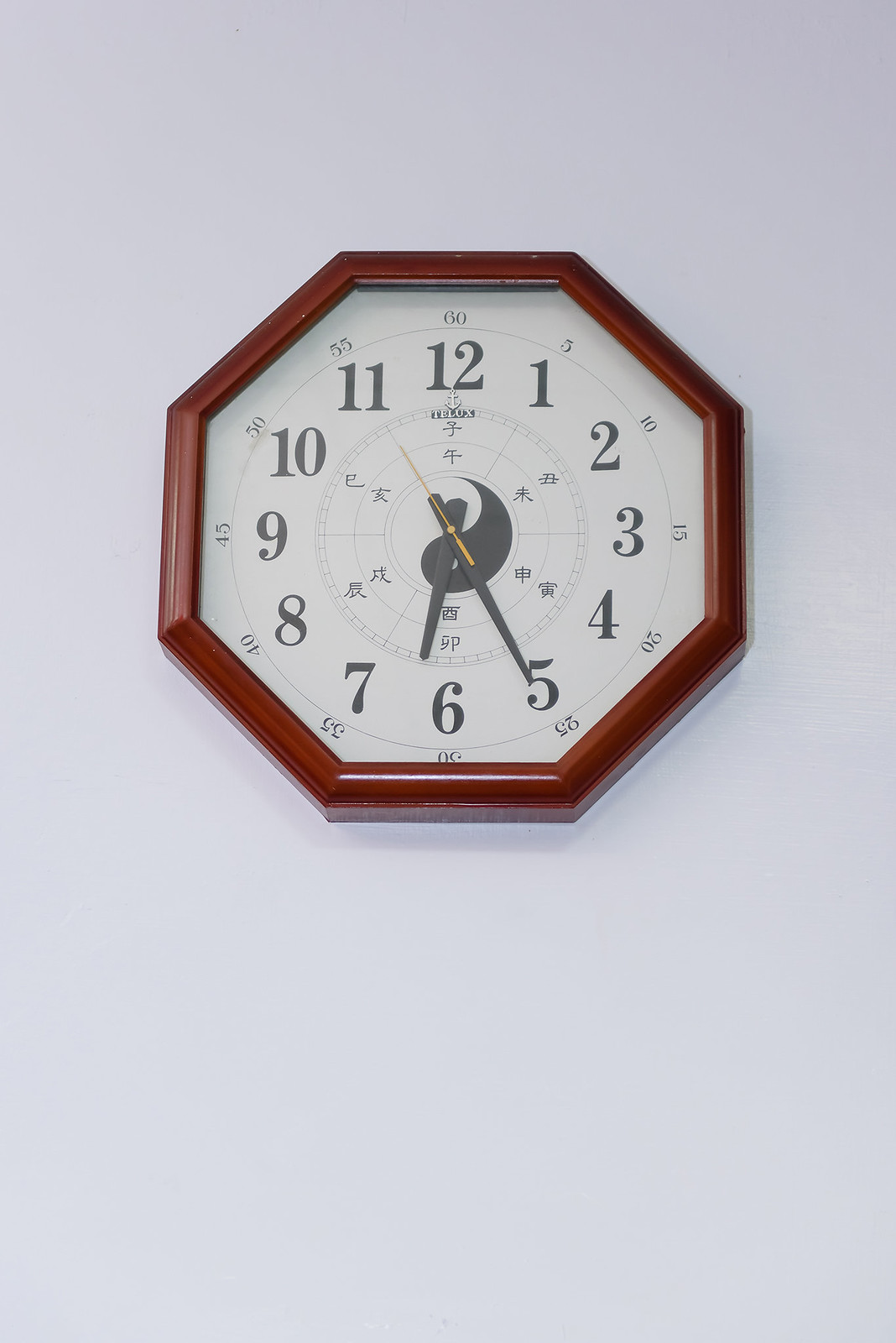This high-quality photograph captures a unique clock that resembles the shape of a stop sign. The clock has a rich, chocolatey-orange hue, giving it an elegant and warm appearance. The white clock face contrasts sharply with its dark, intricate black font, displaying numbers in a clear and legible manner. The clock features two black hands and one distinctive yellow hand, all centered over a striking black teardrop design. The clock is mounted on a pristine white wall, casting subtle shadows that add depth and dimension to the composition.